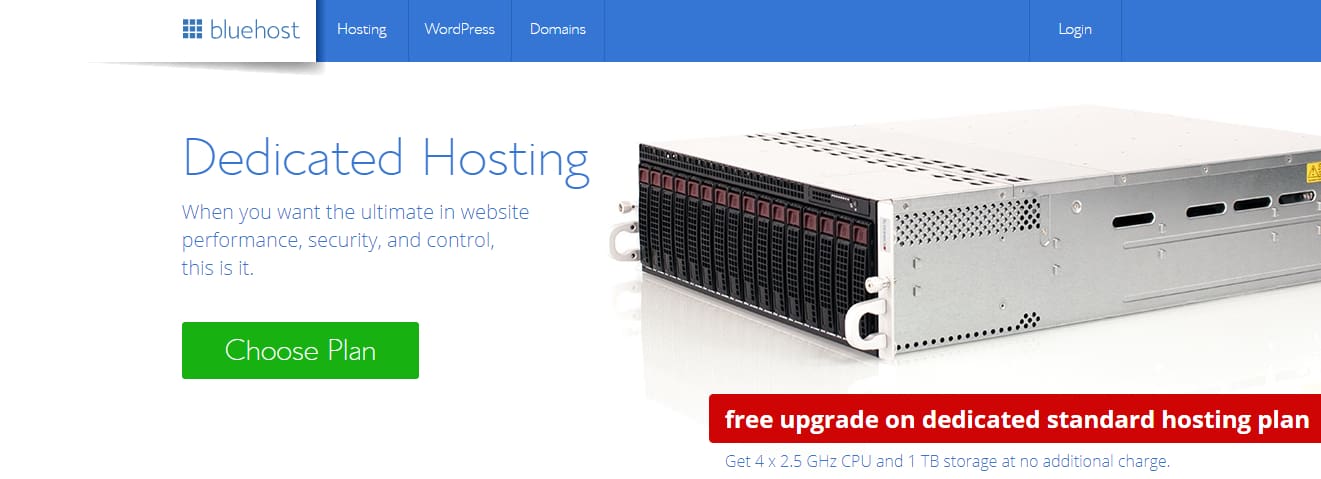The image depicts a partial view of the BlueHost website interface. At the top, against a white background, the BlueHost logo is prominently displayed, consisting of a grid of nine smaller blue squares forming one larger square, accompanied by the text "BlueHost." Adjacent to the logo on a blue strip, the categories "Hosting," "WordPress," and "Domains" are written in white text. Further to the right, the word "Login" is also visible.

Below this header, the background shifts to white and a headline reads, "Dedicated Hosting," followed by the description: "When you want the ultimate in web performance, security, and control, this is it." Directly beneath, there is a green button labeled "Choose Plan" in white text. To the right of the button, there is an image of a computer server, which appears to be a white mechanical unit, resembling a hard drive.

Further down, a red horizontal strip announces "Free Upgrade on Dedicated Standard Hosting Plan," followed by a gray section stating, "Get 4x2.5 GHz CPU and 1 TB storage at no additional cost," highlighting the offer's details.

The overall layout of the image is horizontally extended and only a portion of the full webpage is visible.